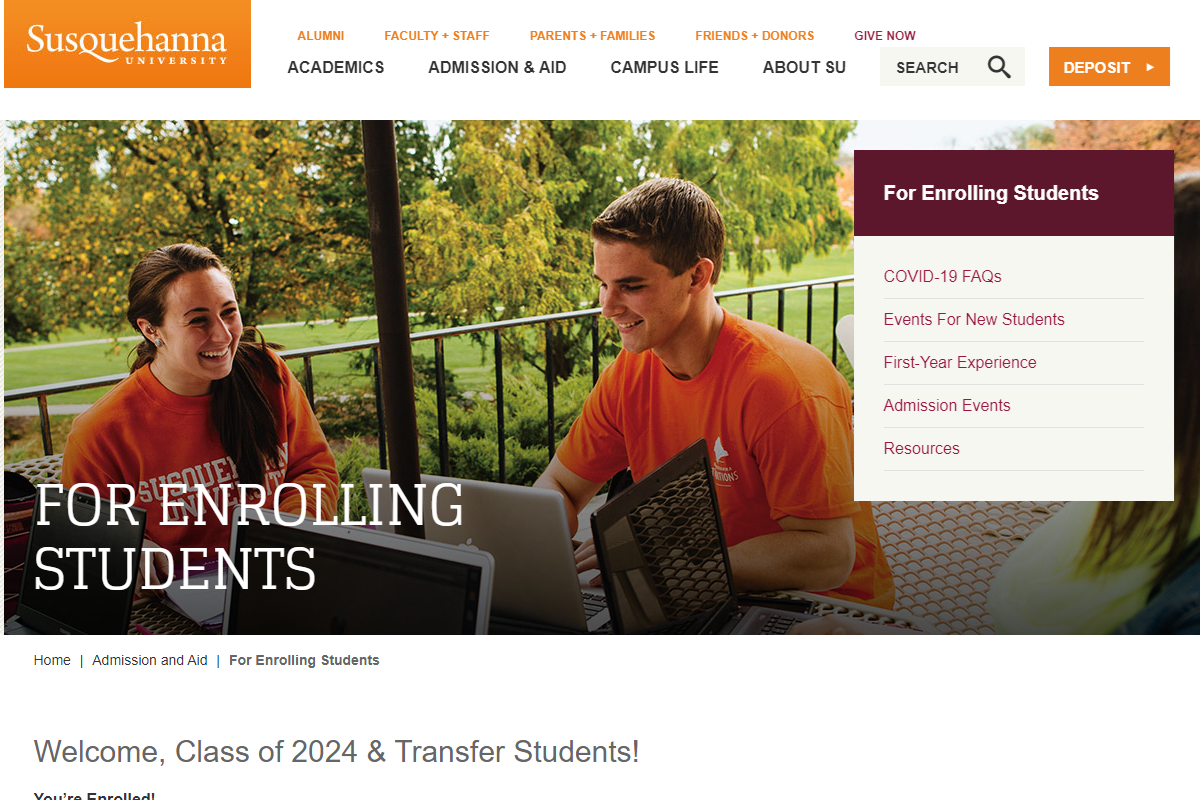The screenshot captures the home page of Susquehanna University's website. Dominating the top left corner of the page, "Susquehanna University" is proudly displayed within an orange rectangle. Spanning the upper section are various navigational elements: categories from left to right, an easily accessible search bar, and a conspicuous "Deposit" button. The focal point of the page is a vibrant photograph featuring two jovial students seated at a table with at least three laptops. The female student on the left and the male student on the right both wear bright orange shirts, and their smiles suggest a welcoming and friendly environment.

To the right of this main image, there is a notable text box titled "For Enrolling Students," accompanied by a drop-down menu that offers topics such as COVID-19 facts, events for new students, first-year experiences, admission events, and additional resources. Positioned at the bottom left of the student photograph, the phrase "For Enrolling Students" is reiterated. Directly beneath this are navigational buttons labeled "Home," "Admission and Aid," and "For Enrolling Students."

The footer of the page contains a welcoming message in large gray text, stating, "Welcome Class of 2024 and Transfer Students." Unfortunately, the lower portion of this message is truncated, but it partially reads, "You're Enrolled." The overall design and layout of the webpage exude a sense of warmth and readiness for incoming students.